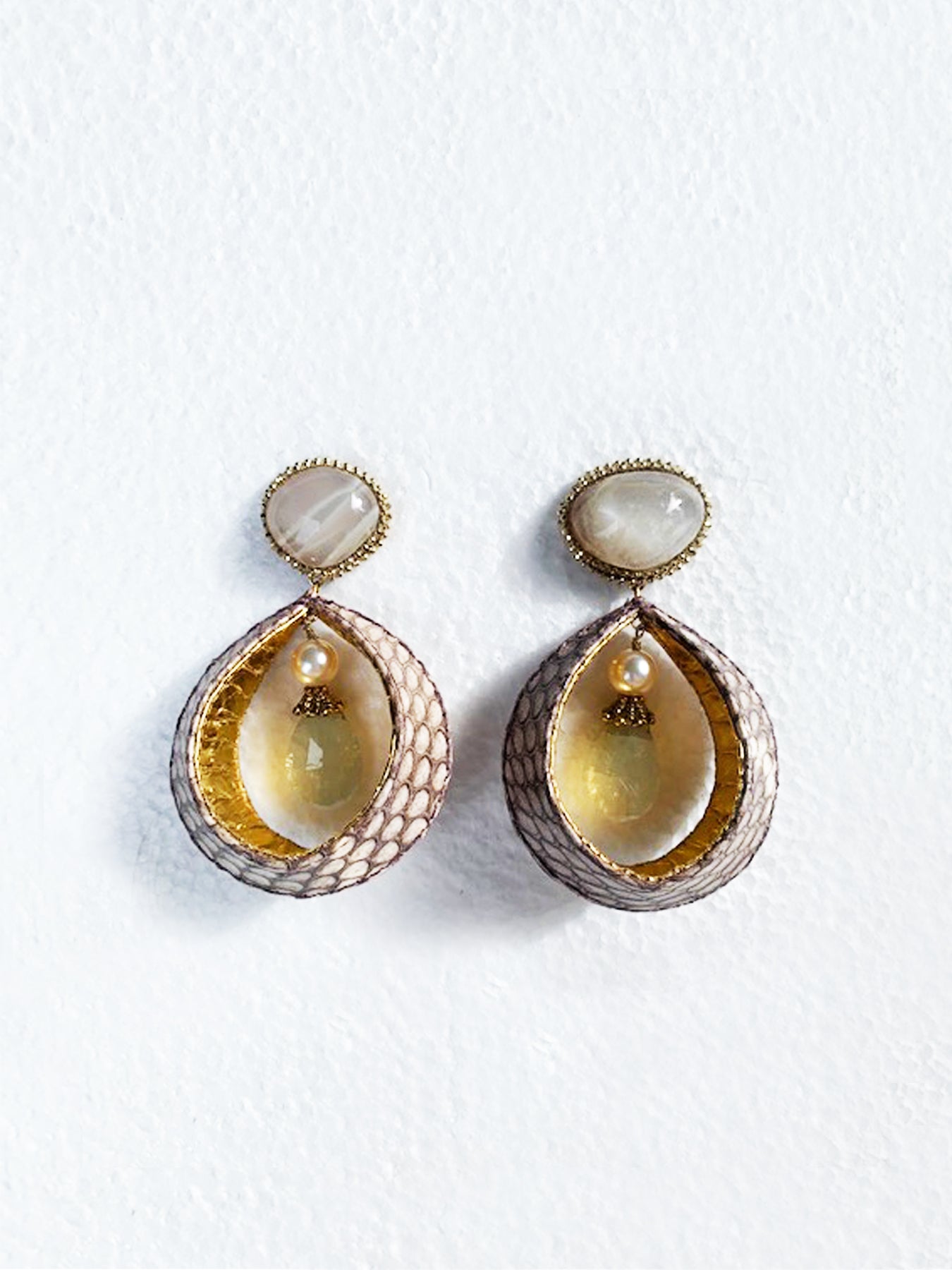This is a photograph of an intricately designed pair of antique-style earrings placed against a white background. Each earring features a pierced stud at the top, framed in a delicate silver prong setting, with a central mother-of-pearl stone. Below the stud, a drop link chain leads to an oval-shaped drop earring showcasing a sophisticated interplay of gold and white in a mesh pattern around its border. The inner section of the oval is purely gold, thickening at the bottom and narrowing at the connecting points. Suspended within the larger oval is a cream-colored drop pearl delicately encased in an antique holder, beneath which dangles a faceted light green gemstone. The overall composition exudes a handcrafted charm, with slight variations hinting they might be uniquely handmade.